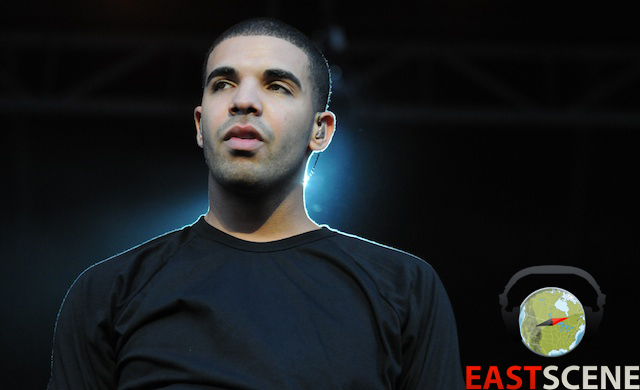This horizontally aligned rectangular image features a man who appears to be a familiar figure, possibly an athlete or actor, although his identity is uncertain. The man, resembling Drake, has almost shaved short black hair and thick black eyebrows. He faces the viewer but his gaze is slightly off to the left, with his head cocked in that direction and his mouth slightly open. He is dressed in a black t-shirt, which appears wrinkled, but the cut-off at the bottom of the image makes it unclear whether it has short or long sleeves. An earpiece is visible in his left ear, suggesting he might be on stage. The background is predominantly black, punctuated with a white light just below his left ear and some blurry metal poles crossing from left to right at the top of the image. A small globe symbol, featuring gray headphones and triangular black and red segments, is located at the lower right-hand corner. Beneath this globe, the text "EAST SEEN" is displayed prominently, with "EAST" in large red letters and "SEEN" in tan or white letters.